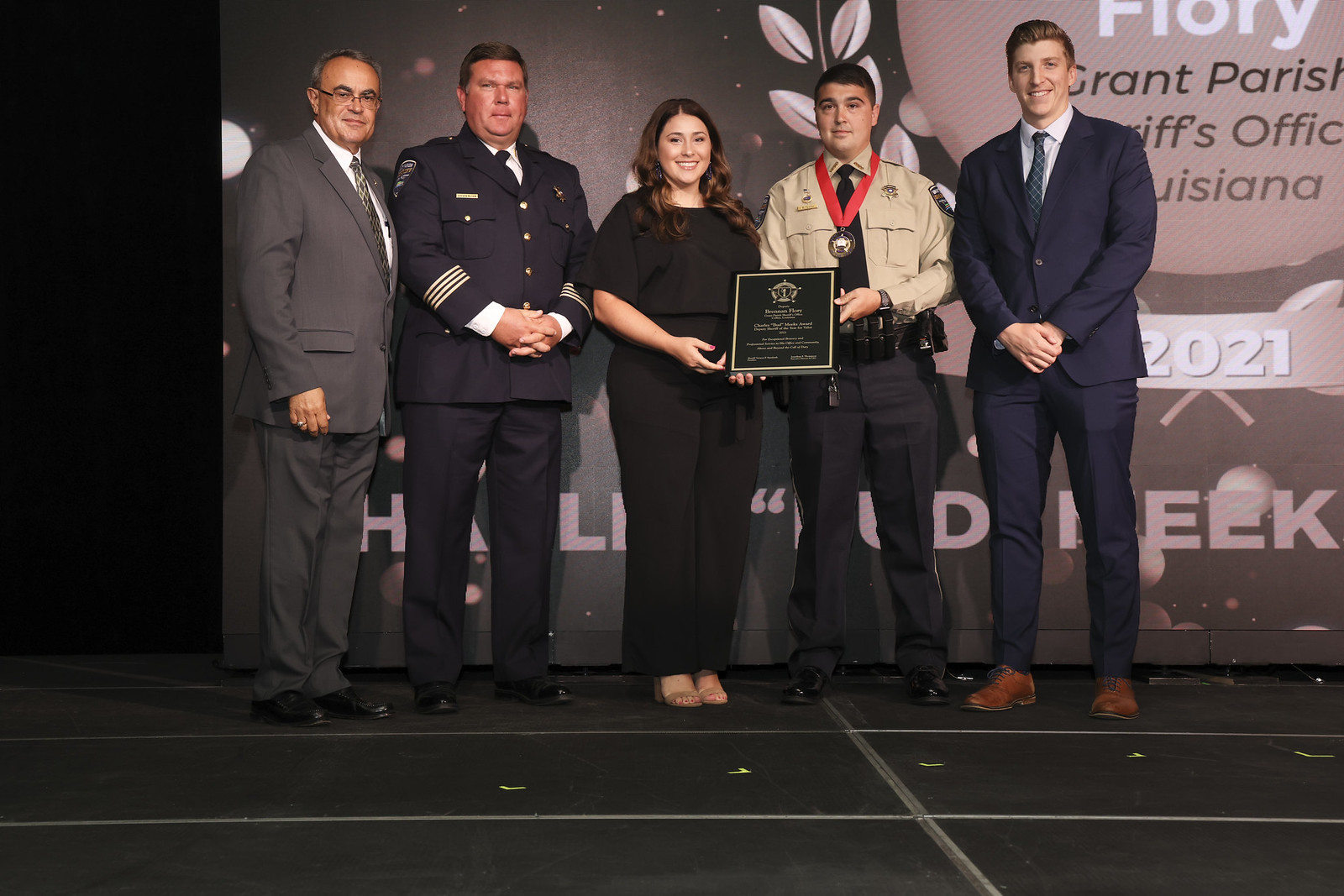In this photograph taken on a stage, five individuals are prominently posed against a backdrop that reads "Grant Parish Sheriff's Office, Louisiana, 2021." From left to right, the first person is an older man in glasses, dressed in a gray suit with a white shirt and gray tie. Next to him stands a middle-aged man in a blue and gold police uniform. The central figure is a woman in a black blouse and pants, with long, curly brown hair and a warm smile. She holds a black and brown plaque, sharing it with a young man beside her. This man, second from the right, is dressed in a tan sheriff's uniform with dark pants and a utility belt. He has dark hair, wears a black tie, and a red ribbon with a medal around his neck. On the far right stands another young man with short blonde hair, dressed in a blue suit with a matching blue shirt and tie. The stage has a black floor and the backdrop’s brown background features the event details. The woman and the man in the blue suit are smiling broadly, while the others maintain more reserved grins.